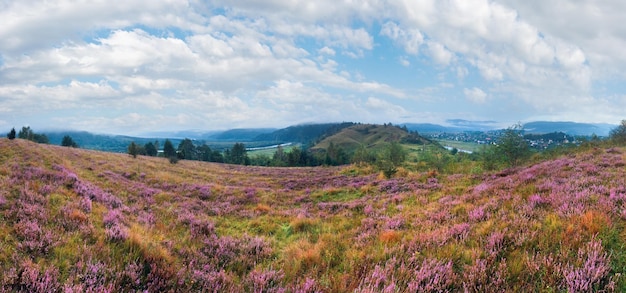The image depicts a picturesque meadow abundant with wildflowers nestled in the Blue Ridge Mountains. The foreground is a vibrant tapestry of dark pink and light purple flowers, interspersed with patches of dry grass. The wildflowers, notably lilac-colored, blanket the field in an untamed beauty, with no signs of agricultural interference. Scattered evergreen trees dot the landscape, adding to its natural charm.

In the background, a series of low brown and blue hills roll gently, reminiscent of the Appalachian and Smoky Mountains, with no snow-capped peaks in sight. These hills frame a distant village, contributing to the scene's serene and rustic allure. Above, the sky dominates the upper half of the image, presenting a canvas of soft blue interspersed with big, fluffy white clouds. The expansive sky adds to the idyllic and timeless quality of the panorama, capturing the tranquil essence of this mountain meadow.